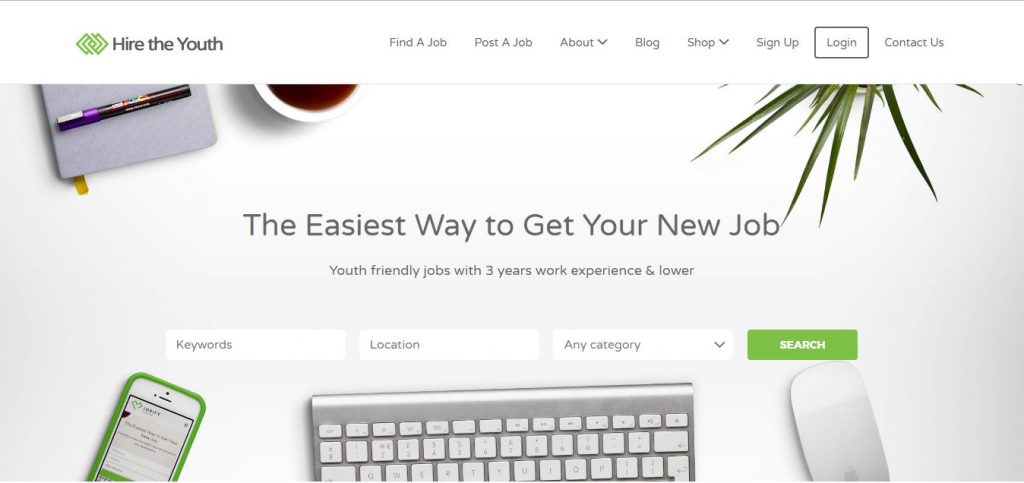The screenshot captures a website interface with several distinctive elements:

At the very top, there's a white rectangular border spanning from left to right. In the top left corner, there's a logo comprising two or three interlinking green squares, with the text "Hire the Youth" in black to the right of it. 

Moving to the right, the top navigation menu features black text links in the following order: "Find a Job," "Post a Job," "About" with a downward-facing caret next to it, "Blog," "Shop" also with a downward-facing caret, "Sign Up," "Login" enclosed in a black rectangular box, and "Contact Us."

Below this navigation bar, the background image shows a white desk setup. On the left side of the desk, there's the bottom part of a gray book with a black pen laid horizontally across it. Adjacent to this, there's a white coffee cup filled with brown coffee. 

On the far right, some slender, pointed leaves of a green desk plant are visible. Towards the middle bottom of the image, there's a silver Mac keyboard with white keys. Next to the keyboard on the left, a smartphone with a green case is visible; its screen displays what appears to be the Hire the Youth website. To the right of the keyboard, a white Mac wireless mouse is placed.

In the middle of the page, a bold black text states, "The easiest way to get your new job." Below in smaller black font, it reads, "Youth-friendly jobs with three years work experience and lower." 

Further down, there are three white rectangular selection boxes. The one on the left is labeled "Keywords" in a dark gray font. The middle box is labeled "Location," and the rightmost box says "Any Category" with a downwards-facing drop-down arrow. To the right of these boxes, there's a green rectangular button with the word "Search" in white centered in it.